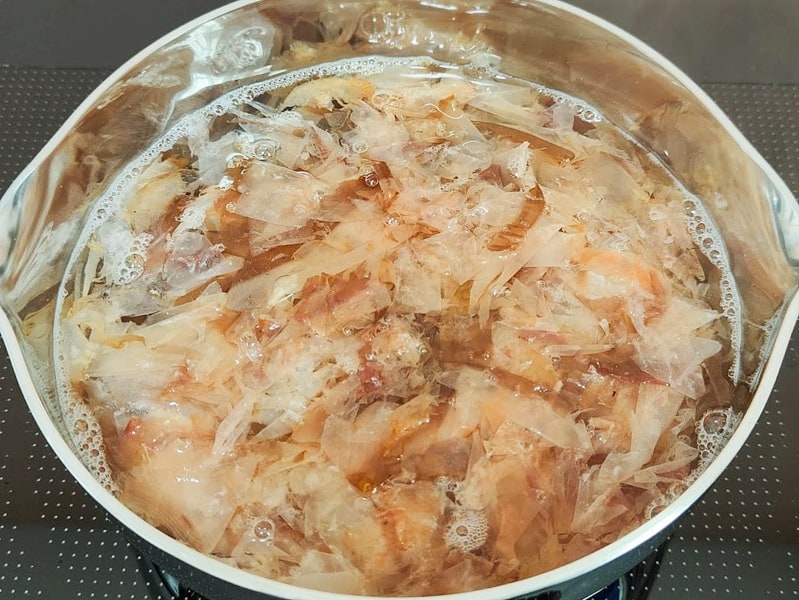This color photo, taken indoors, provides a zoomed-in view of the interior of a cooking pot, likely placed on an induction stove. The pot, which appears to have a ceramic or green exterior and a shiny metal interior, showcases boiling liquid that may be water or a light broth. The liquid contains numerous fine, thin pieces of ingredients, possibly onions or wonton paper, exhibiting shades of cream and light brown. A foam forms around the edges, suggesting the beginning stages of cooking. The pot's silver rim is partially visible, featuring small bubbles indicative of the cooking process. Though the exact contents are somewhat mysterious, they could include onions, shrimp, potatoes, cabbage, or even fish, contributing to what might be a soup or stew. The pot also features spout-like extensions, hinting at its design for easily pouring out its contents.